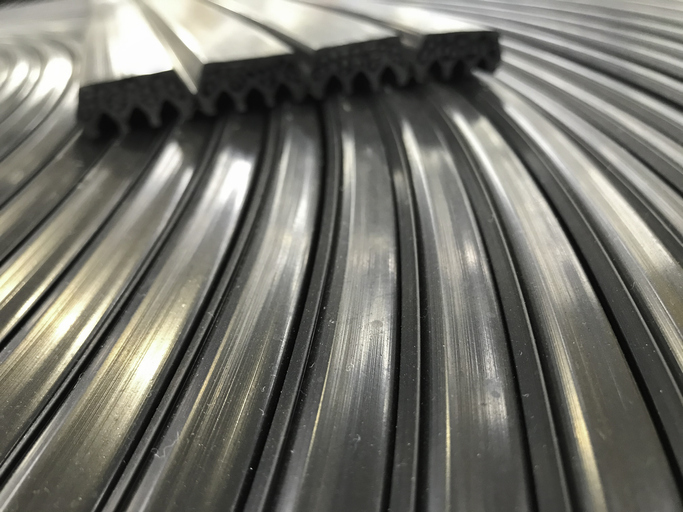The image depicts a set of four metal bars situated on a metal runway. The bars, which appear to be lawn rails or some form of structural component, are aligned toward the back and left of the runway. Each of the metal bars features three notches at their base, where they make contact with the runway; these notches have a shape reminiscent of Monopoly houses, rising straight up before tapering to a pointed cone. The bars seem either closely positioned or potentially connected to one another. The runway itself has distinct metal striations or tracks, though there is no visible mode of transportation, suggesting that the bars might simply slide across it. Scattered across the tracks are small bits of dust and debris. Meanwhile, the background includes an out-of-focus, curved metal object with concentric circles and indentations, potentially a cleaning tool. The overall scene is illuminated by a light source, highlighting the brushed metal finishes and subtle details, including bits of lint on the bars.